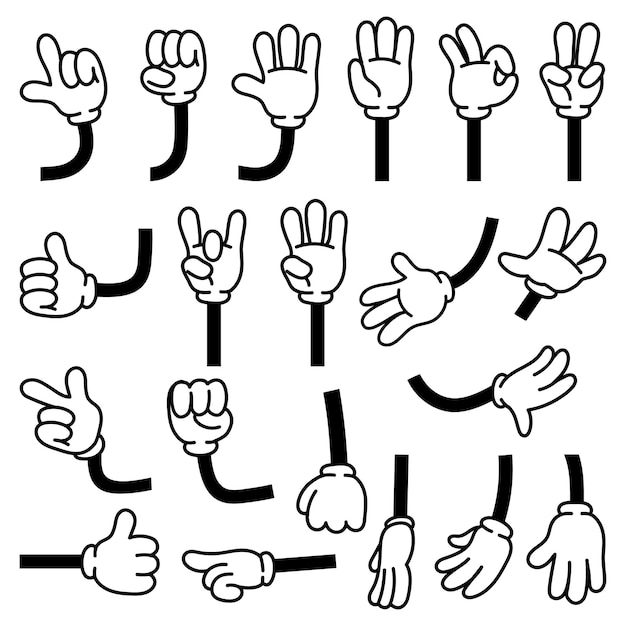The image depicts a variety of cartoon-like white-gloved hands, each attached to a black strip representing an arm, reminiscent of Mickey Mouse’s hands. The hands are arranged in several rows, displaying around 20 to 25 different hand gestures, which appear to be a guide for sign language letters. Each hand has three fingers and a thumb, and they are shown in multiple poses from various angles. The gestures include a mix of familiar signs such as a peace sign, an okay sign, a thumbs up, a devil sign, and a rock sign. Some hands are fully open, some are half-closed, and others form fists with the thumb either curled into or wrapped around the fingers. There are also single-finger points and multi-finger configurations, all designed to illustrate distinct shapes and motions for clarity and comprehension.